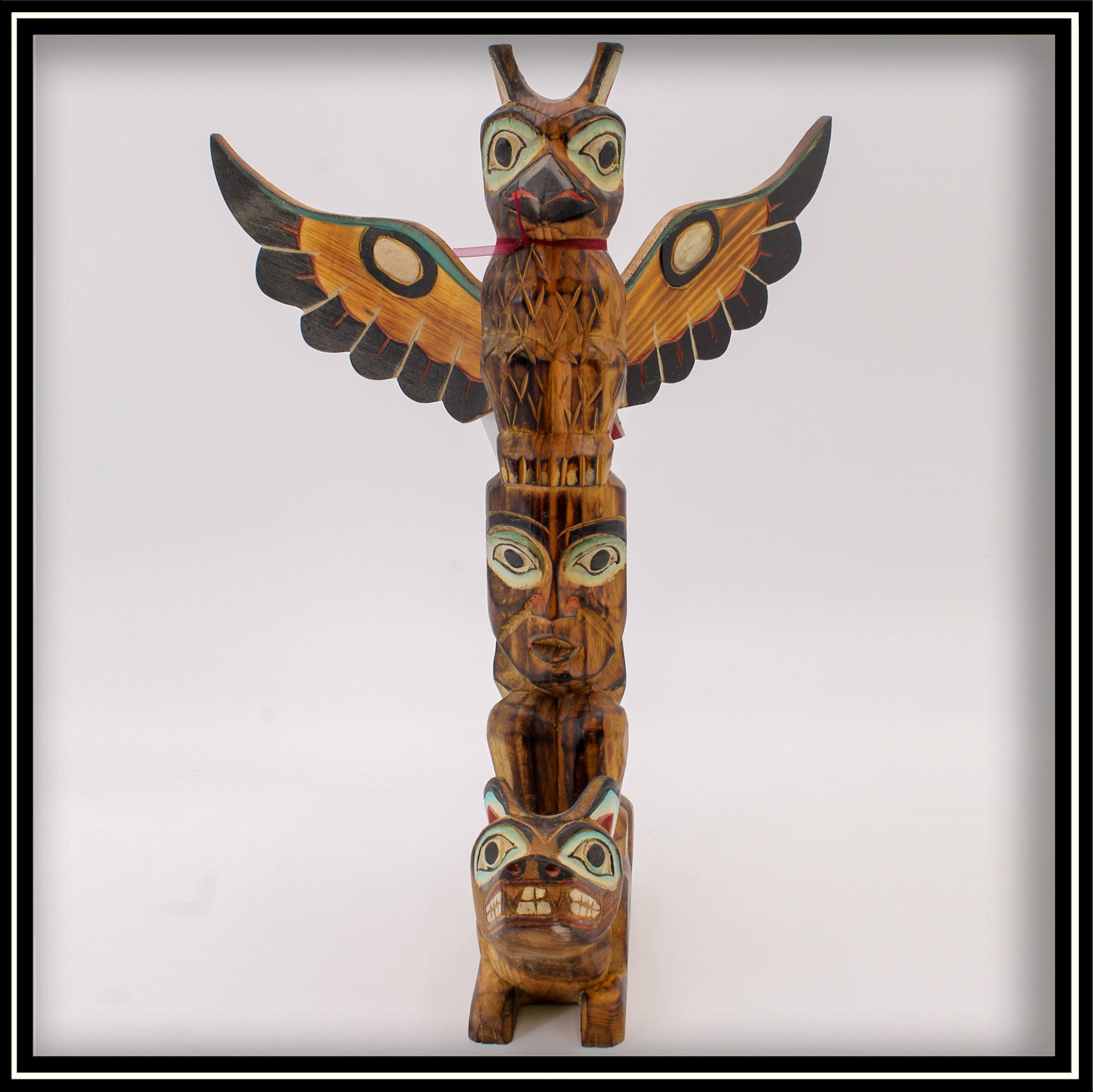This photograph features a beautifully hand-carved and hand-painted totem pole set against a very light gray background and framed by a multi-layered border: a thick black outer border, a thin white middle border, and another thick black inner border. The totem pole, crafted from dark orangish-black wood with more orangey and brown tones on the outside and darker inner wood, is composed of three distinct characters.

At the base of the totem pole, there is a dog-like creature with eyes outlined in aqua blue and white, almond-shaped with large black pupils. The creature's ears are pointy and feature a red triangle at the center, surrounded by white and aqua blue.

Above this base creature is a humanoid face with unpainted lips, striking blue almond-shaped eyes with thick, arching black eyebrows. The figure has a thin nose and a slightly open mouth, adding to its expressive demeanor.

Crowning the totem pole is a bird, likely an owl, characterized by an X pattern carved into its chest. It boasts a black beak accented with red in the opening, large almond-shaped eyes similar to the other figures, and blocky ears sticking out at angles. The spread wooden wings of the bird feature white and black circles, outlined with blue on top, black tabs with red lines in the center, and pointy black tabs at the tips.

This intricately detailed totem pole is not just a decoration piece but a stunning representation of craftsmanship, combining vibrant colors and intricate carvings to bring each character to life.